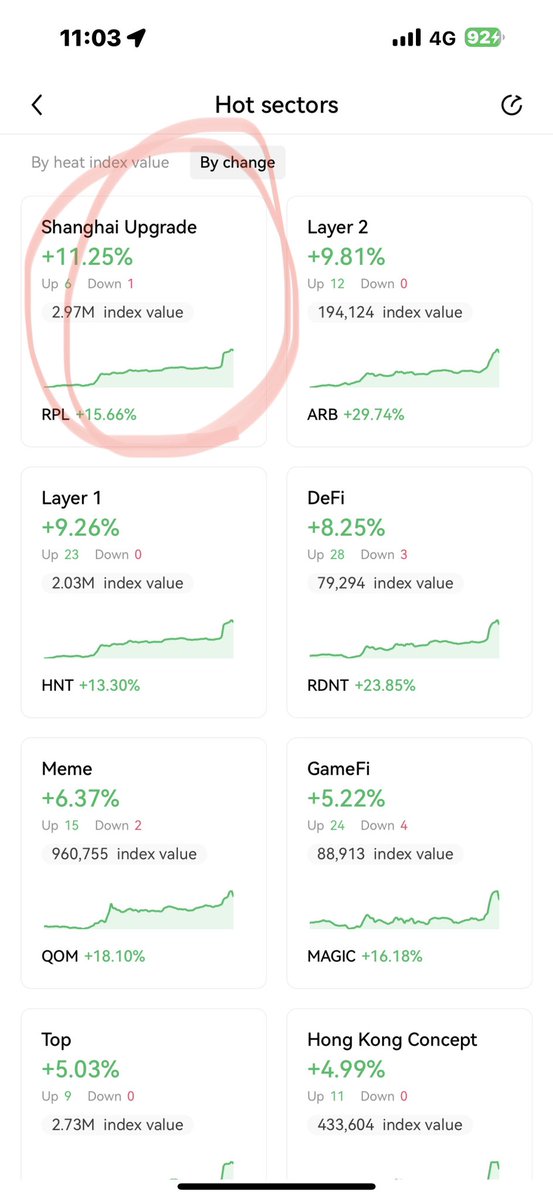The image depicts a screenshot taken on an iPhone displaying specific information about various sectors. In the top left corner of the phone's screen, the time is shown as 11:03. Adjacent to this, the location services icon indicates that the device's location is enabled. Moving to the top right section, the network signal strength is at its maximum, displaying 4 out of 4 bars, alongside the 4G connectivity icon. Notably, the battery percentage is critically low at 2%.

The main content of the screenshot highlights various sectors and their performance metrics:

1. "Hot sectors, sought by heat index value,"
2. "By change, Shanghai upgrade plus 11.25%,"
3. "Top 6 down 1,"
4. "2.97 million index value,"
5. "Layer 1 plus 9.26%, up 23, down 0,"
6. "Defi plus 8.25%."

These details outline the significant indexes and percentage changes, including notable statistics of sectors such as Shanghai, Layer 1, and Defi.